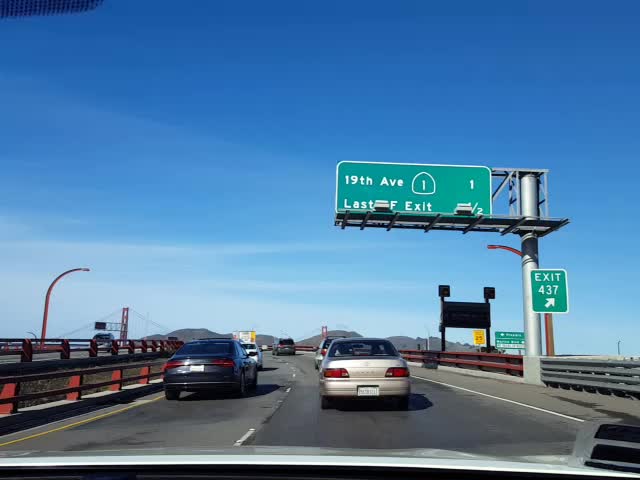The image, taken from inside a moving vehicle, shows a view through the front windshield of a notable interstate highway. The scene is dominated by a gradient sky, transitioning from a light blue at the horizon to a striking dark blue at the top of the frame, with a thin sheet of cloud cover present on the left side. This road, which may be part of the Golden Gate Bridge or a similar cable-stayed bridge, features two lanes filled with several vehicles, including a black sedan in the left lane and a silver sedan in the right lane.

On the left side of the frame, the image captures a large metal beam extending upward, supporting a green sign with white lettering indicating "19th Avenue" and "Exit 437" with an arrow pointing right. A distinct red guardrail on the left contrasts with the initially metallic then red-tinted guardrail on the right. Further in the background, additional green and yellow signage is visible, albeit too distant to read clearly. The presence of streetlights and distant hills enrich the backdrop, adding to the depth and complexity of the scene. Silver poles, creating triangular structures, add to the architectural interest of the bridge setting, completing this dynamic and picturesque highway snapshot.